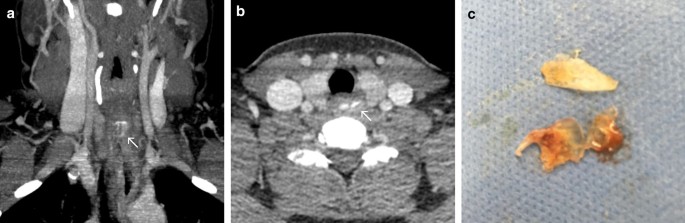This series presents three square images labeled A, B, and C in the upper left corner of each frame. Images A and B are black and white, resembling x-rays, with small arrows indicating points of interest. Image A showcases a vertical structure running from top to bottom, with the arrow highlighting white smears and spots at its center. Image B features a more rounded central area, with the arrow pointing to a diminutive white bump. In contrast, Image C diverges by displaying a colored image with a reddish-brown and cream composition, possibly depicting biological material smeared on a piece of open-weave surgical cloth. This final image includes an arrow, though it seemingly points at nothing discernible.